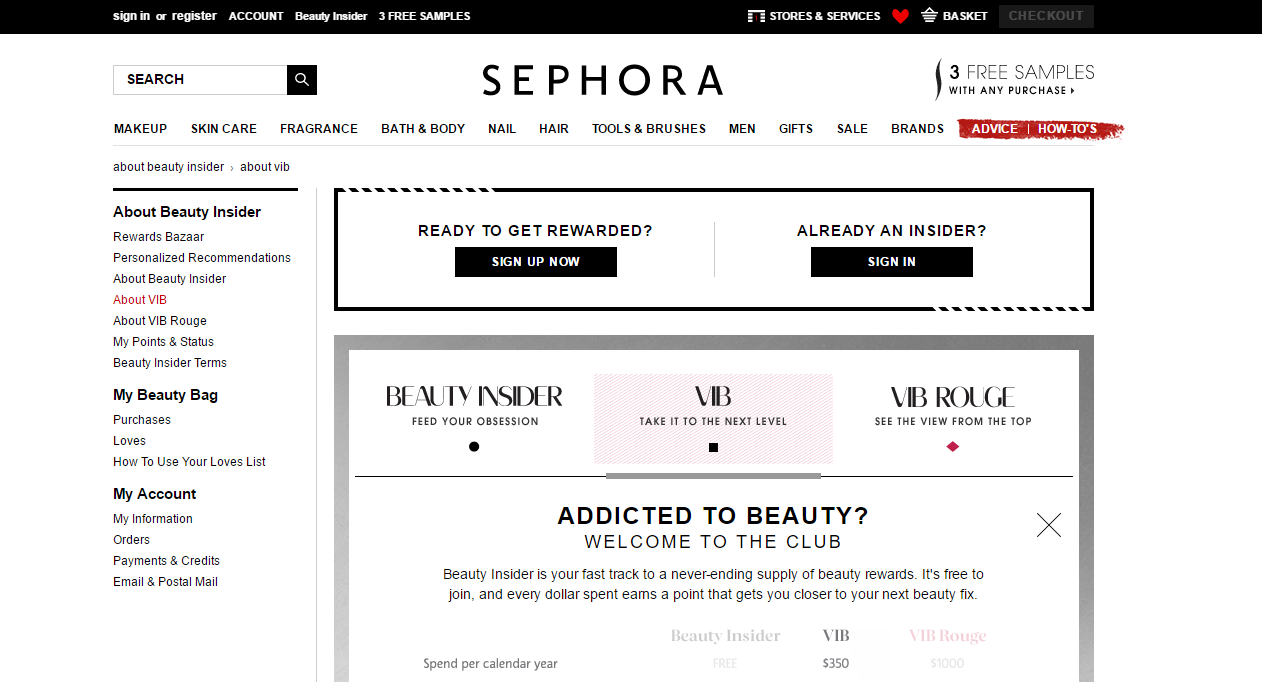This is a detailed description of an image depicting a Sephora website's webpage. 

---

The image showcases a webpage from the Sephora website. Dominating the top middle of the page is the prominent "Sephora" logo. To its left is a search box accompanied by a black search button, inviting users to input their queries. To the right of the logo, the text "three free samples with any purchase" is displayed.

Above these elements lies a sleek black toolbar that extends across the entire top of the page. On the far left of this toolbar, clickable links include "Sign In or Register," followed by buttons labeled "Account," "Beauty Insider," and "Three Free Samples." On the far right segment of the toolbar, you'll find links for "Stores & Services," a red heart icon, the word "Basket" accompanied by a basket icon, and the grayed-out link "Checkout."

The main body of the webpage features two prominent buttons at the top. The first button indicates, “Ready to get rewarded,” with a black "Sign Up Now" button beneath. Adjacent to this, a prompt reads, “Already an Insider?” followed by a black "Sign In" button.

Additionally, a large pop-up menu takes center stage with the message, “Addicted to beauty? Welcome to the club.” To the left of the page, another menu serves as a navigation toolbar, directing users to sections like "Beauty Insider," "My Beauty Bag," and "My Account."

Overall, the webpage is meticulously organized, combining functional navigation elements with promotional content, inviting users to explore and engage with various features and offers.